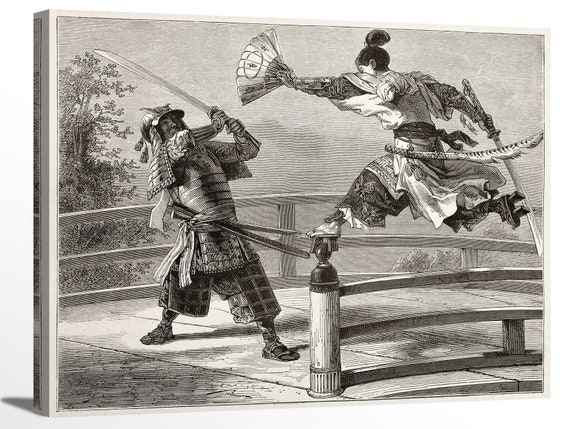This detailed black and white pen and pencil drawing, elegantly framed in a thin wooden frame, depicts a dramatic duel between two warriors. Dominating the scene is a samurai knight clad in traditional samurai garb, complete with a large helmet and a protective breastplate. He stands poised for attack, gripping a sword raised high above his head. His attire includes distinctive black and silvery checkered pants, and he sports open-toe sandals. Opposite him, perched on a fence, is an opponent dressed in flowing white robes adorned with dark designs. This figure, with hair styled in an intricate kabuki bun, wields a fan in one hand and a sword in the other, wearing platform-style wooden sandals with thick heels. The backdrop features a mountainous landscape to the left, with a solitary tree reaching up to a gray, moody sky, setting the stage for their battle on a bridge. The intricate details and traditional Japanese aesthetic underscore the intensity of the confrontation captured on canvas.